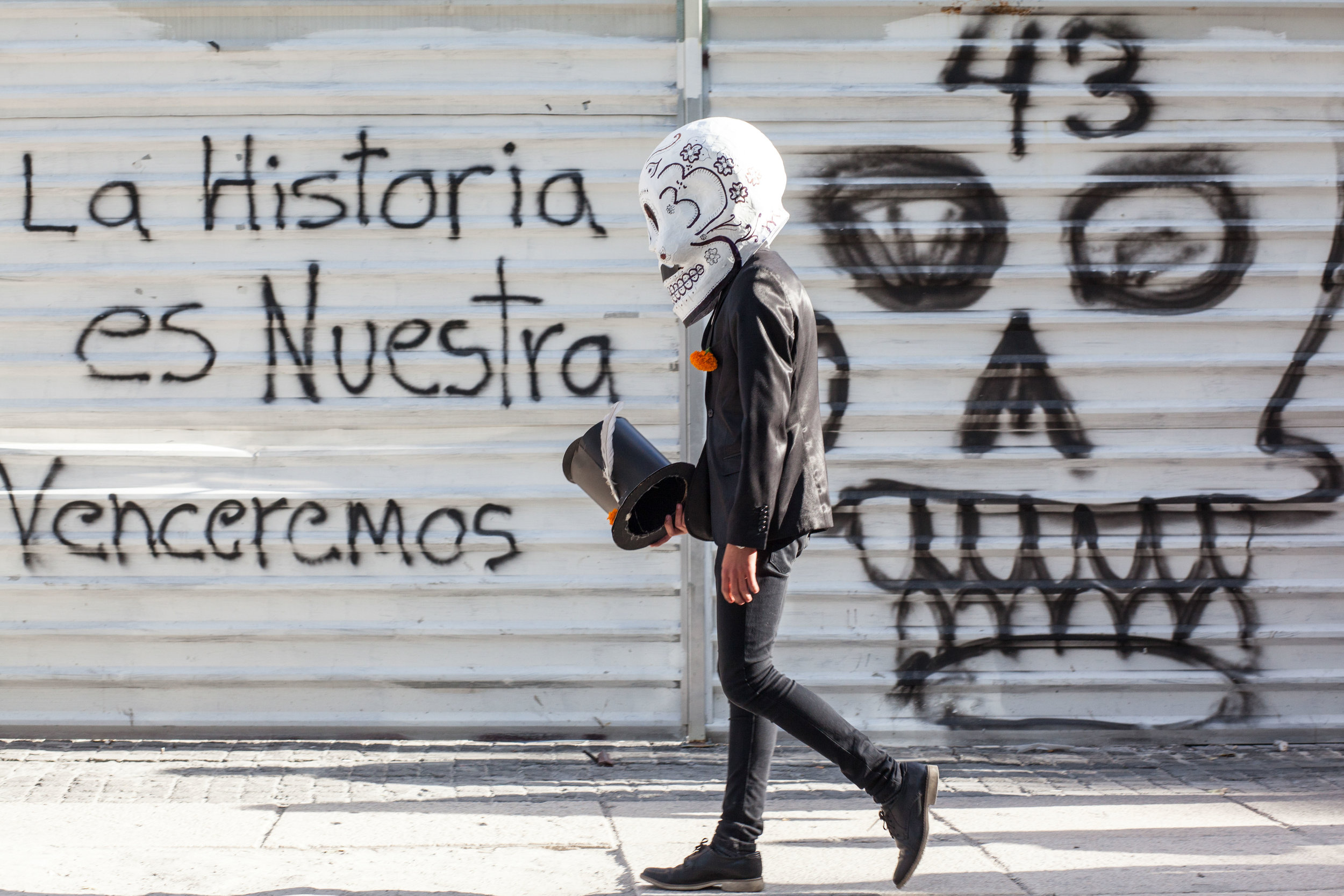In the image, a thin individual dressed in all black is walking down a light-colored cement sidewalk, appearing to be somewhere in Mexico or South America. They are wearing a black leather jacket and dark-colored pants, complemented by dark gray tennis shoes. The figure's right hand holds a tall black top hat, while the left arm hangs naturally at their side. On their head, they sport a striking white skull helmet, which appears to be a repurposed motorcycle helmet with painted black eyes, nose crevices, and teeth detailing; small painted flowers adorn the sides, enhancing its eerie appearance.

The backdrop is a white fence or corrugated metal wall adorned with graffiti. On the left side of the wall, it reads in bold black letters, "La Historia es Nuestra Venceremos," a Spanish phrase suggesting a historical or triumphant message. To the right of these words, the wall features an intricately drawn skull with the number "43" prominently displayed on its forehead. The skull graffiti, achieved with black spray paint, depicts hollow eyes, a nose cavity, and a row of teeth, further emphasizing the skull motif carried by the individual walking past.